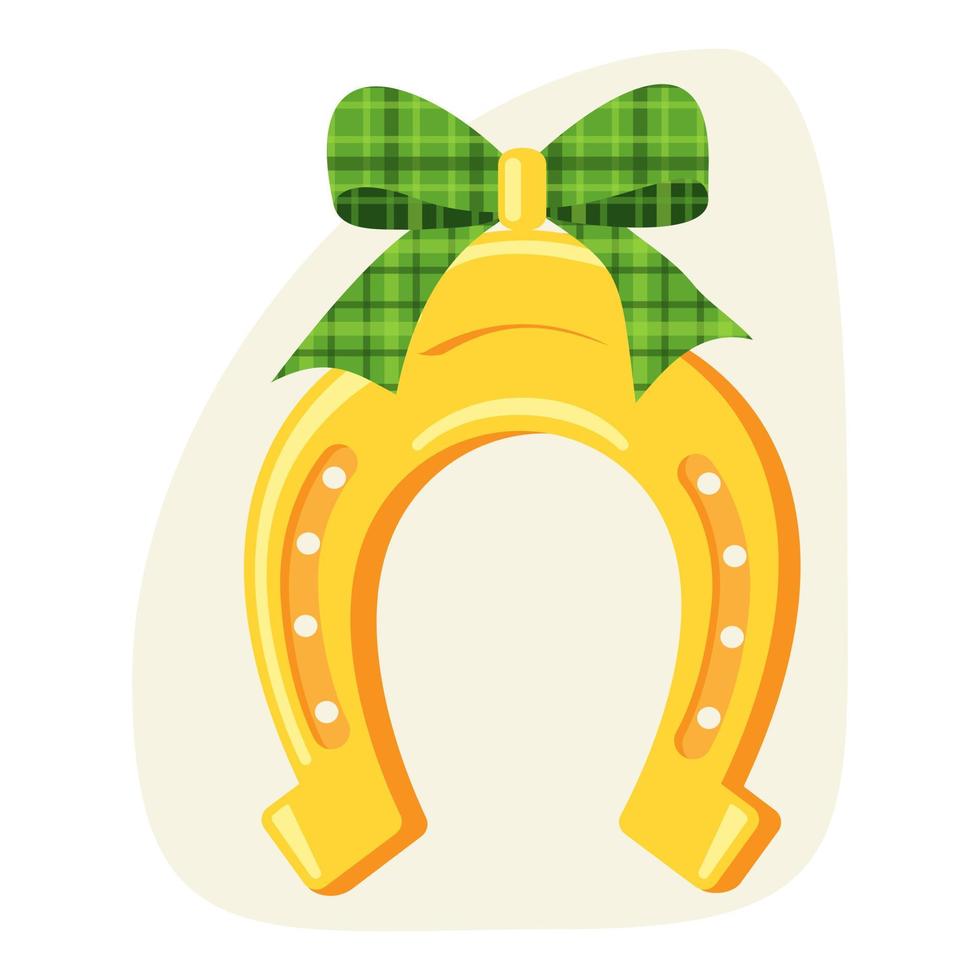In the image, a detailed pixel art showcases a vibrant yellow horseshoe with orange trim along the shaded edge. Each side of the horseshoe features a long groove filled with a darker orange hue and adorned with four white dots. Atop the horseshoe sits a bell-shaped ornament crowned with a green plaid bow, which appears neatly integrated into the structure. The entire scene is set against an irregular, roughly triangular gray background with rounded points that curves to accommodate the horseshoe's shape. The image is accentuated by a crisp white backdrop, adding a clear and clean visual distinction to the vibrant colors and intricate design, evoking a sense of luck, possibly referencing St. Patrick's Day.